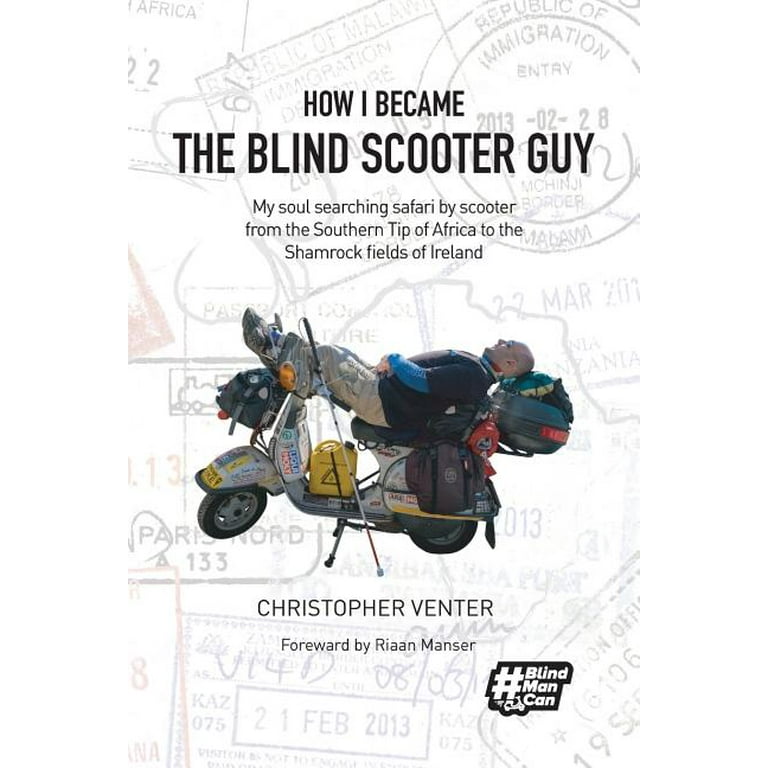The image appears to be the book cover for "How I Became the Blind Scooter Guy: My Soul Searching Safari by Scooter from the Southern Tip of Africa to the Shamrock Fields of Ireland" by Christopher Venter, with a foreword by Riaan Manser. The background features a collage of passport stamps, providing a black and white, postcard-like aesthetic that signifies the author's travels, including an entry dated February 28, 2013, suggesting a border crossing. Dominating the foreground is a striking photograph of a heavyset, clean-shaven man reclining on a silver scooter, with his feet draped over the handlebars and his head cushioned by a gray storage container at the back. The scooter has black and gray wheels and a yellow gas can affixed to it. The man is dressed in a black t-shirt over a blue long-sleeved shirt, khaki pants, and sneakers. His white cane lies alongside him, symbolizing his blindness and the journey he undertook. The bottom-right of the cover includes the phrase "#BlindManCan" next to a white and black scooter symbol, reinforcing the theme of overcoming adversity through adventurous travel.